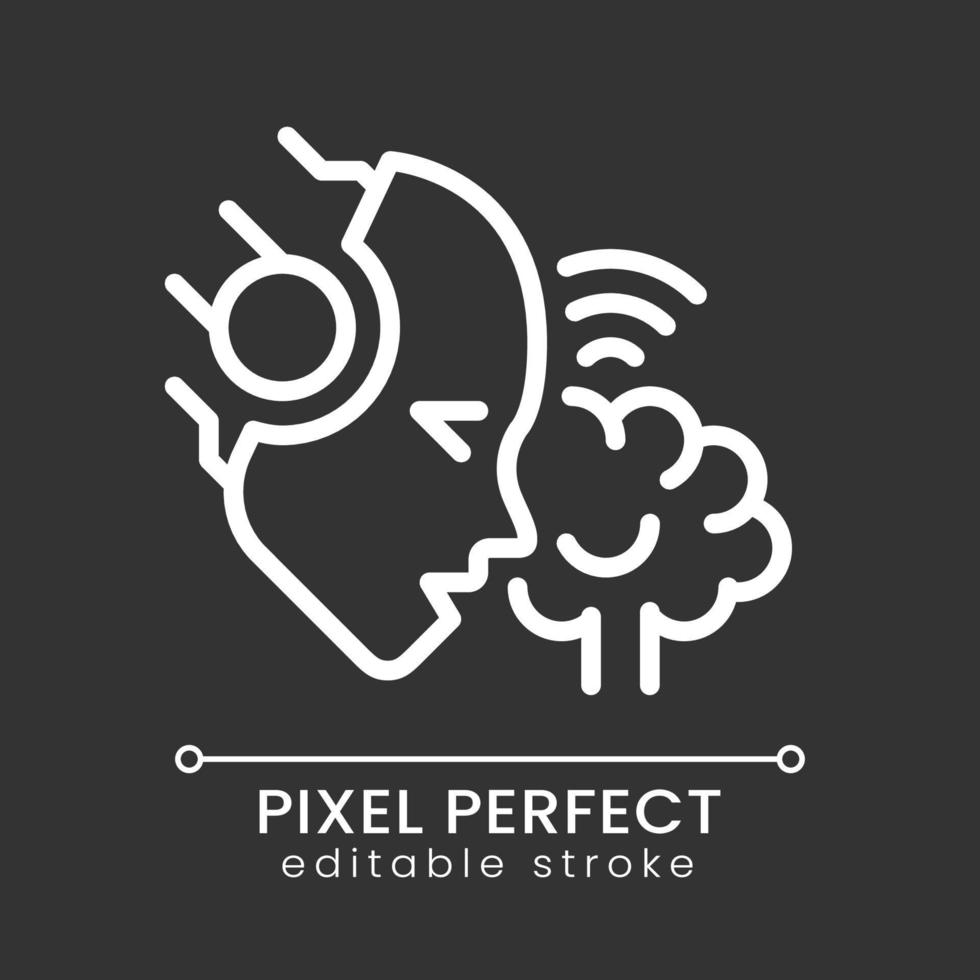The image is a logo with a square shape, featuring equal-length sides and a solid dark gray background. At the top center, there is a prominent white graphic depicting a humanoid robot head in a side profile, looking towards the bottom right. The robot's head features a circle where the ear should be and lines extending from the back, enhancing its mechanical appearance while mimicking human features. To the right of the head, there is a round white cloud with three curved lines emerging from it, resembling a Wi-Fi signal. A white line separates this graphic from the text below. The text, also in white, reads "PIXEL PERFECT" in all caps on one line and "editable stroke" in all lowercase letters beneath it.